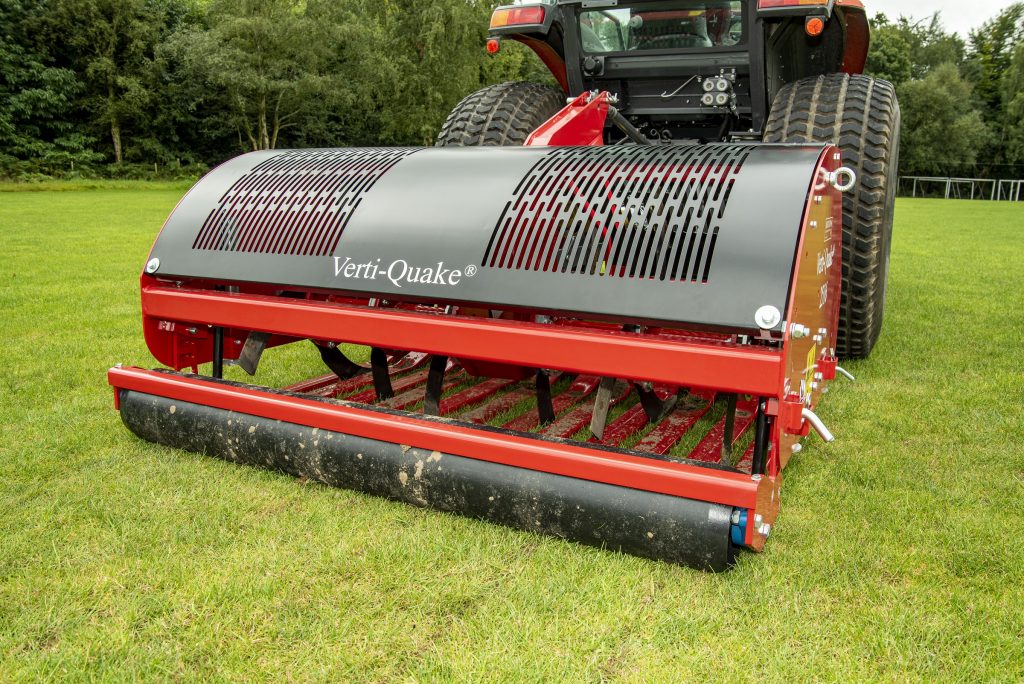The image depicts a large piece of farm machinery, likely used for tasks such as mowing or pressing down grass. The vehicle, manufactured by Vertiquake, prominently displays its name on the central front portion. It is characterized by its bright red and black colors and features two enormous visible wheels; additional wheels are likely present but not visible in the image. The machinery has a significant front attachment, consisting of what appears to be blades or rollers, designed to exert pressure on the ground or carry out fieldwork. The vehicle's body incorporates materials that might include plastic or glass, with grilles on top providing ventilation. Positioned in an expansive, well-tended field of healthy green grass, the scene includes some divots in the ground near the front of the machine. In the background, there are dense clusters of trees situated at a distance from the open field, emphasizing the large and uncluttered workspace.